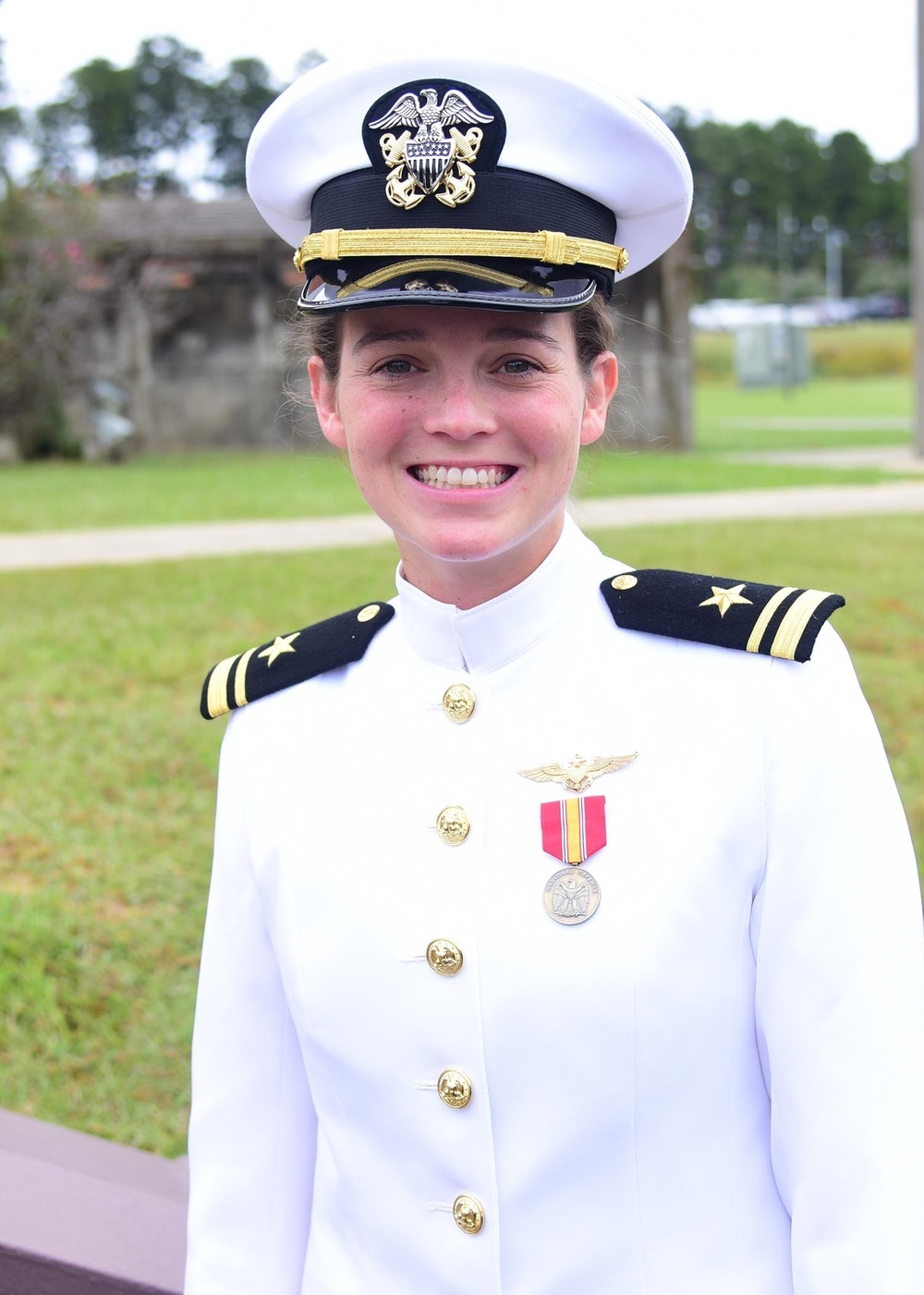In this vertically aligned outdoor photograph, a young Caucasian woman, an ensign in the United States Navy, stands smiling in the foreground. She is dressed in her formal dress white uniform, featuring a long sleeve jacket decorated with several round gold buttons down the front and shoulder patches that are navy blue with gold stripes and a star. She also wears a badge on the right chest, which consists of a gold medallion with an eagle over a red-and-yellow-striped ribbon, as well as a sea warfare pin and a single ribbon. Her naval hat, characterized by a white top, black rim, gold ribbon, and an eagle emblem, sits neatly on her head with her brunette hair tucked underneath, highlighting her brown eyes.

The background of the image showcases a well-manicured, low-cut grassy field interspersed with several concrete pathways. An older-looking, dark gray building with several windows and a maple tree with blooming flowers stands behind her to the left. Additional smaller concrete monuments are scattered around. Further in the distance, a cluster of trees completes the serene outdoor setting. The scene looks slightly overcast, providing a muted light that does not cast strong shadows, and the blue sky suggests a calm day.